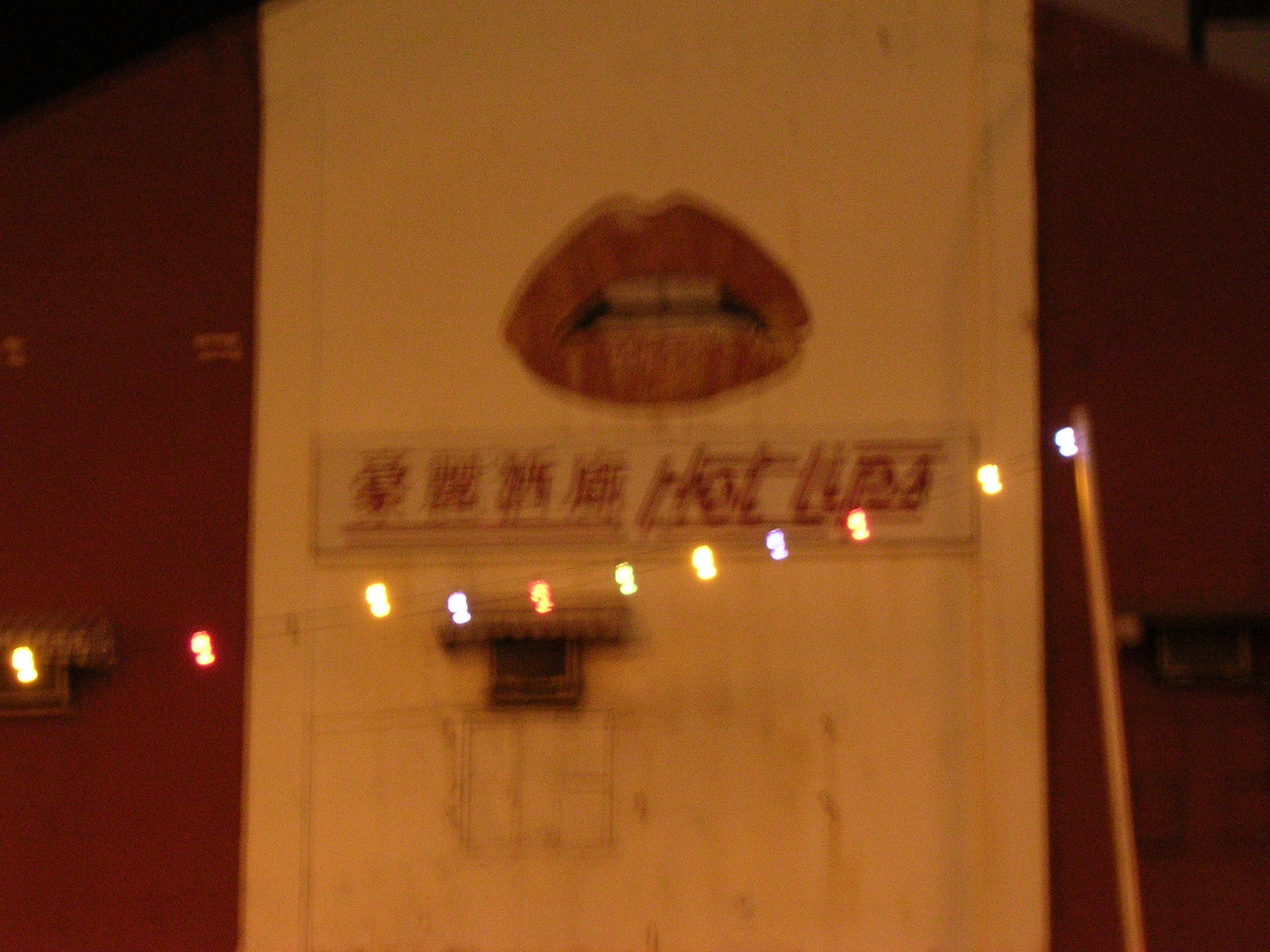This landscape orientation photograph, despite being slightly blurry with noticeable motion blur, captures a vibrant nighttime or low light scene. Dominating the center of the image is a towering yellow wall adorned with a striking graphic of large, red lips baring white teeth. Beneath this eye-catching artwork, there's text that adds context to the scene. To the left, four Chinese characters can be seen, while to the right, the words "Hot Lips" are just discernible, suggesting the wall belongs to an establishment named "Hot Lips", potentially a club or business. Adding to the lively ambiance, a strand of colorful Christmas lights hangs festively in front of the yellow backdrop, enhancing the visual appeal of the scene.